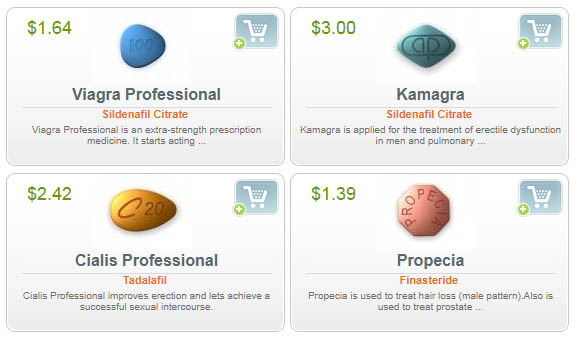The image depicts a promotional arrangement of four different pills offered by a pharmaceutical company, highlighting Viagra Professional, Chemagra, Cialis Professional, and Propecia. Each pill is represented within its own rectangular section of the image. In the upper left-hand corner of each rectangle is the price, marked in green text, listed as $1.64. 

In the center of each rectangle, there is a visual representation of the corresponding pill. Below the image of the pill, there is a button featuring a white shopping cart icon set within a gray box, accompanied by a green plus sign, indicating an option to add the item to the cart.

The name of each pill is prominently displayed in bold text, followed by its official pharmaceutical name in red print. Additional brief descriptions provide more details about each medication. For example, the section for Viagra Professional notes "Sildenafil Citrate" and describes it as an extra-strength prescription medicine that starts acting quickly, though the detailed description trails off with ellipses.

The layout is consistent across all four sections, creating a clear and informative visual summary of each product:
1. Viagra Professional
   - Sildenafil Citrate
   - Described as an extra-strength prescription medication.
2. Chemagra
3. Cialis Professional
4. Propecia

Each product is accompanied by succinct pharmaceutical information, enhancing the viewer’s understanding of the medication's purpose and characteristics.